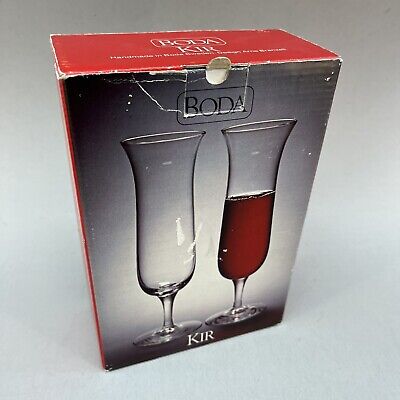This image features an old, beat-up cardboard box against a light gray background. The box, which appears to have housed two wine glasses, displays a worn and dented facade with a few rips and tears, indicating its age. The front of the box is designed with a grayish background that includes a white burst effect. Prominently featured at the top is the word "Boda" in black, while the bottom displays "K.I.R." in white. The box also shows two tall, tulip-shaped wine glasses. The glass on the left is empty, highlighting its elegant fluted shape, while the glass on the right contains a red liquid, possibly tea or wine. The top of the box is red with white text that repeats "Boda Kir," accompanied by a smaller, indecipherable white sentence. The sides of the box, which are partially visible, also appear to be red, reinforcing the antiquated and well-used nature of the packaging.